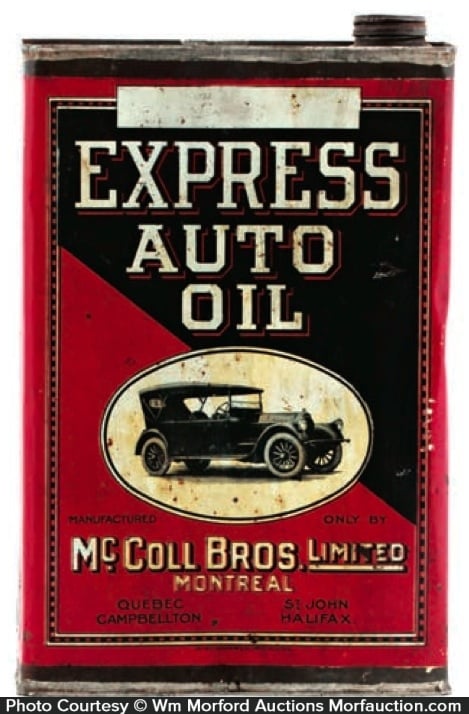This is a detailed photograph of an antique, rectangular-shaped oil can labeled "Express Auto Oil." The can predominantly features a red and black color scheme, with the upper right section being black where the primary text stands out in bold white letters. The inscription "Express Auto Oil" is prominently displayed on the black part. There is a white oval with a black border in the center of the can, containing an illustration of an old black car, likely a vehicle from the 1920s or 30s. Below the illustration, additional text reads, "McColl Brothers Limited, Montreal," indicating the manufacturer’s origins in Montreal, Quebec, and St. John's, establishing its Canadian roots. The can, which has a rusty appearance and shows signs of age, features a small, tin, screw-on spout at the top right corner. The entire setup rests on a white background, highlighting the can's colors and text. The bottom of the photograph includes a watermark that states, "Photo Courtesy of W.M. Morford Auctions," with the website morfauction.com noted for attribution.